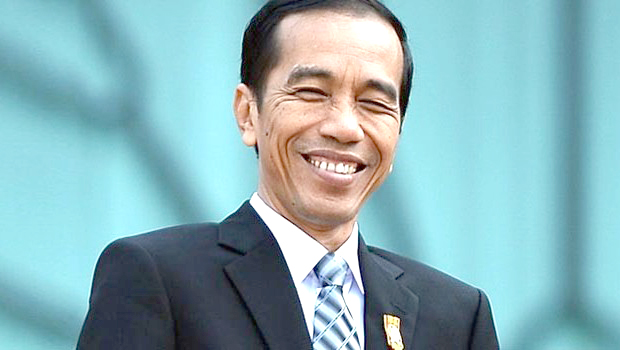This rectangular, landscape-oriented photograph captures a man of Asian ethnicity, possibly Indonesian President Joko Widodo, standing from the chest up. He is dressed in a black suit adorned with a gold pin on the left collar, a white collared shirt, and a blue and white striped tie. The man has short, dark hair and is beaming widely, his eyes squinted shut, revealing his teeth in a very noticeable way. The backdrop is a light blue color interspersed with dark blue, almost black, lines, likely a banner or stage decor, suggesting a formal setting.